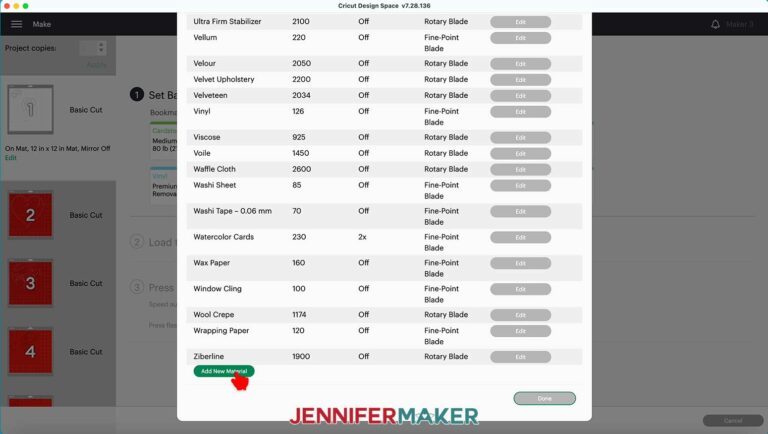This image is a screenshot of the Cricut Design Space application, specifically version 7.28.136, as indicated at the top center. The screenshot displays the application running on a Mac OS platform, identifiable by the red, yellow, and green dots located in the top left corner of the window. Cricut Design Space is an interface for users of Cricut devices, which are tools designed for cutting various materials to create arts and crafts.

At the center of the screen, a prominent white box lists multiple material options for designing with a Cricut device. Each row in this list features the name of a different material, such as ultra firm stabilizer, vinyl, and waffle cloth. Next to each material name, additional details are provided. For example, the entry for vinyl includes the number 126, the state "off," and specifies the use of a fine point blade, which is the appropriate blade for cutting vinyl. 

To the right side of each row, there is a gray oval button labeled "Edit" which allows users to modify the information about that specific material. At the bottom left of the white box, there is a green oval button with the text "Add New Material," accompanied by a red hand silhouette icon indicating the action to add a new material.

Additionally, the bottom center of the image features a logo for Jennifer Maker, with "Jennifer" in red text and "Maker" in blue text. This identifies the creator of the image as Jennifer Maker, a known name in social media.